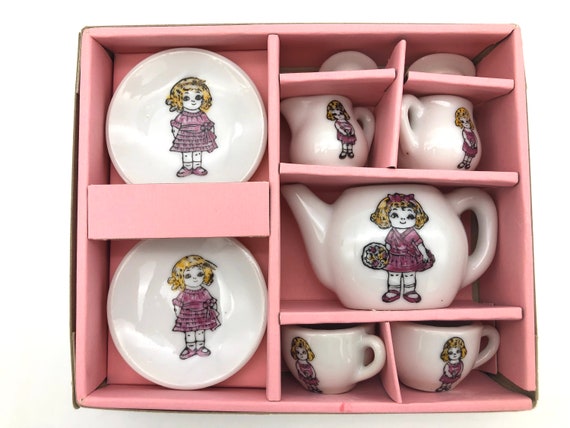The photograph features a child’s tea set neatly arranged in a pink, segmented cardboard box with a white background. The box, although slightly warped from misuse, contains various porcelain items, all adorned with the drawing of a cheerful little girl with short, curly blonde hair and a distinctive ruffly pink dress. The set includes two small white saucers positioned on the left side of the box; each depicts the girl standing with her arms behind her back, white ankle socks, and pink Mary Janes.

In the upper section, there are two small pitchers meant for cream and sugar, each featuring the girl with her hands in front of her. Positioned centrally is a white porcelain teapot that shows the girl smiling, looking towards the right, with a pink bow in her hair, and holding a bouquet of flowers in her right hand. Below the teapot are two smaller teacups, also adorned with the image of the girl, this time clasping her hands in front of her waist without the pink bow in her hair. The entire set is uniformly white and glazed, creating a cohesive and charming tea set ideal for imaginative play.